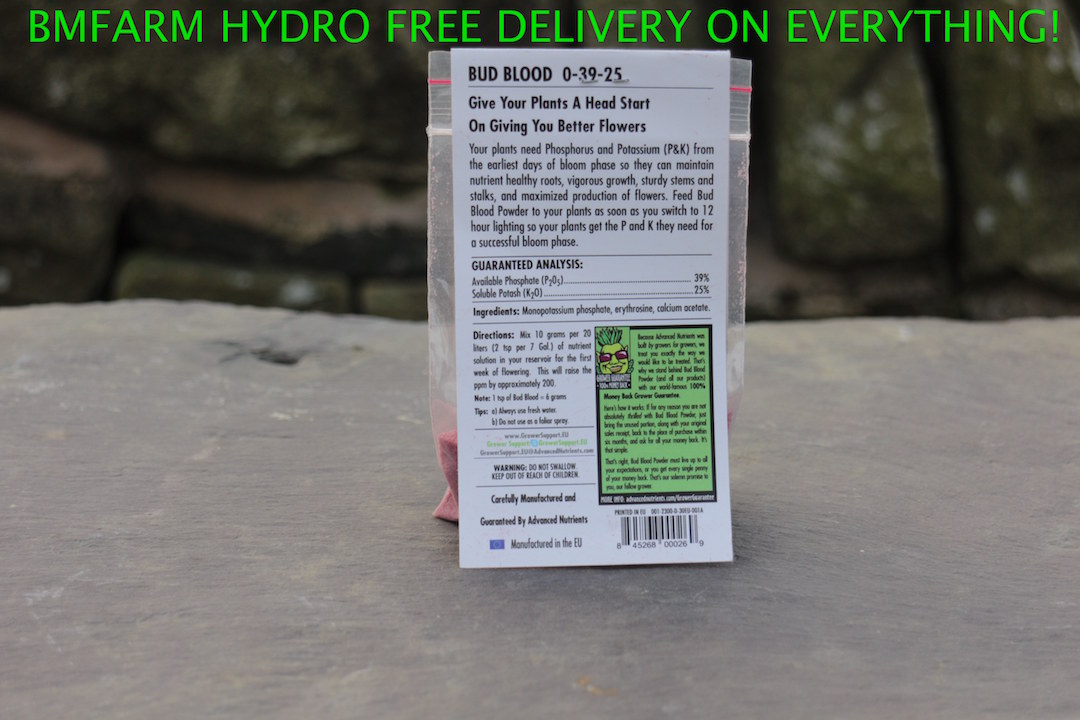In the image, we see a small, light gray concrete wall outdoors, with a zippered plastic bag containing a red powder. The bag is partially obscured by a detailed label stapled to it. The label, which has a white background with black text and a distinct green text area, prominently features the product name "Bud Blood" and a description promoting its benefits for plants. The text emphasizes that Bud Blood provides essential phosphorus (P) and potassium (K) from the early bloom phase, ensuring healthy roots, vigorous growth, sturdy stems, and maximum flower production. Instructions advise feeding Bud Blood powder to plants when switching to 12-hour lighting for a successful bloom phase. There is also a green text box with a cartoon character resembling a vegetable wearing sunglasses, but the text within this area is not fully legible. The top of the label bears the logo "BM Farm," along with a mention of "Hydro free delivery on everything." Additionally, the label includes phrases like "O-39-25" and a money-back guarantee, contributing to the overall marketing message. The barcode is located at the bottom right corner of the label. The image clearly presents Bud Blood as a flower-enhancing product meant for plant nutrient management.